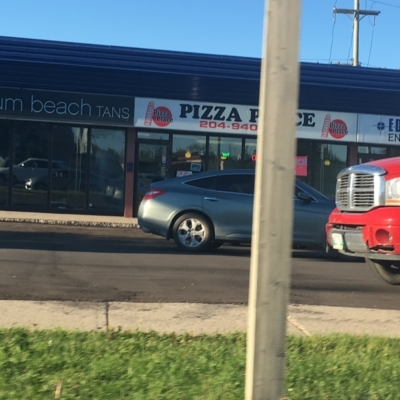This image captures a bustling strip mall scene from across a black asphalt road with two-way traffic. In the immediate foreground, a pale wooden post stands in a fringe of green grass, partially obscuring the view. A concrete sidewalk borders the grass, and adjacent to it is the road where a red truck, likely an SUV, is approaching from the left, and a metallic silver sedan is moving from right to left. Across the street, another sidewalk lines a series of storefronts. On the left, a tanning salon named "Beach Tans" is identifiable by its distinctive green square display. Next to it, a pizza place is marked by a white rectangular sign and a partially visible phone number: 204-940. To the right of these, another business sign is indistinct. Above the buildings, a pale blue sky is visible, with a telephone pole and its network of wires extending into the upper right corner of the frame.